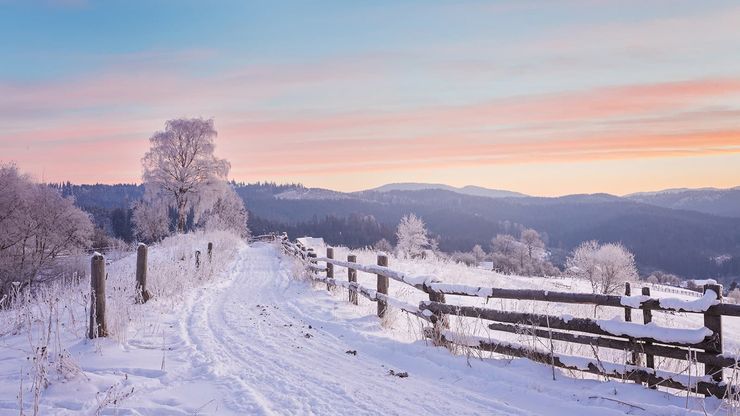This color photograph, captured in landscape orientation, depicts a serene, snow-covered country lane. The trail, which serves as a horse path, lies unplowed with ridges formed by past traffic. Along the right side of the lane runs a split-rail wooden fence, while the left side features only periodic wood posts with wire fencing in between. Snow blankets the ground, accumulating on the horizontal wooden pieces of the fence, and coating the scene in a thick layer of white, while brown lumps of horse droppings can be seen scattered along the path's center.

Clustered around the scene are bare trees heavily laden with snow, creating a picturesque, frost-laden winter wonderland. Further into the distance, the landscape transitions to rolling, forested hills also covered in snow, with larger mountains looming beyond them. The sky is a slate gray typical of a cold winter day, but near the horizon, it gives way to muted tones of pink and orange from the setting sun, intermingling with streaks of horizontal clouds in pink and blue hues.

The peaceful yet cold atmosphere pervades the scene, a reminder of nature’s quiet beauty in the depths of winter. Weeds line the left side of the trail, adding a touch of ruggedness to the otherwise pristine landscape, as the entire vista unfolds with a sense of representational realism.